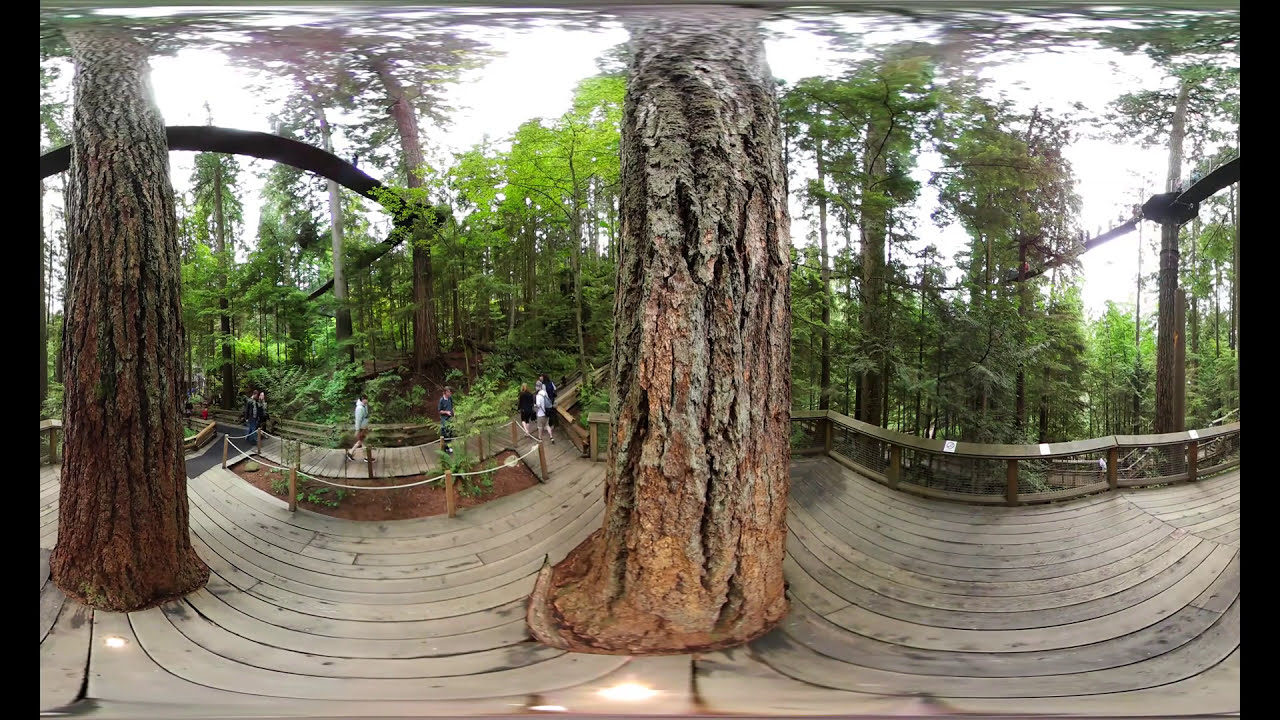In this daytime photograph taken outdoors, we observe a scenic park or nature trail enveloped with greenery. The image, slightly blurred at the top, presents tall trees with vibrant green foliage and tree trunks that transition from light brown to gray as they rise. The trees' texture is distinctly visible, particularly in two prominent trunks positioned centrally and to the left. 

A well-constructed wooden decking area, featuring soft brown planks, curves around these trees, creating a picturesque walkway that guides visitors down a gentle slope. The walkway is fortified with railings, ensuring safety as people traverse this elevated trail. The sky, a soft light blue, peeks through the top of the image, contrasting nicely with the verdant canopy.

Several casually dressed individuals, wearing t-shirts and shorts, meander along the decking. They are distributed throughout the left side of the image, and one appears to be accompanied by a dog. The entire scene is framed in a way that may distort straight lines, resembling the effect of a fisheye lens. This composite view captures the serene beauty and inviting ambiance of a forested park, enveloping visitors in nature's tranquility.